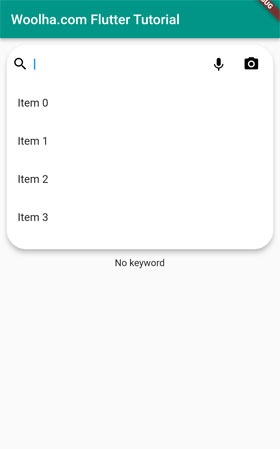This image is a screenshot taken from a cell phone displaying a tutorial associated with the website Wolha.com. Dominating the upper portion of the screen is a green rectangular bar that stretches the full width of the display. Within this bar, "Wolha.com Flutter Tutorial" is prominently featured in white text.

Just below the green bar, there's a large white rectangle occupying most of the screen space. On the upper left side of this white area is a small search icon, accompanied by a microphone icon for voice search and a camera icon for image-based search.

Further down, the screenshot lists four items: "item zero," "item one," "item two," and "item three," but no further details are provided next to these entries, indicating the search yielded no specific results. At the very bottom of the screen, small black text reads, "no keyword," suggesting that the search input may have been either empty or unrecognized.